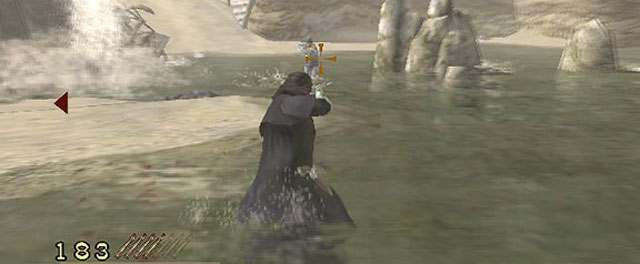The image is a detailed screenshot from a video game, showcasing a character centrally positioned and partially immersed in greenish water. The character is clad in a long black robe and hood, with a small pad extending over their shoulders. Above the character is an orange crosshair, slightly to the right, aiming towards another figure in lighter colors who is standing at a distance, also in the water. Surrounding the scene are large rocks protruding from the water and a small island to the left of the main character. The background features additional water bodies and stone formations against a predominantly beige backdrop. At the bottom left corner of the screen, the number "183" is displayed next to images of arrows, likely indicating the player's remaining ammunition or lives. Additionally, a triangular back arrow, brown in color, is visible in the middle left section of the screen, suggesting a control or navigational element. There are splashing waves both around the characters and in the upper left corner, contributing to the dynamic water setting.